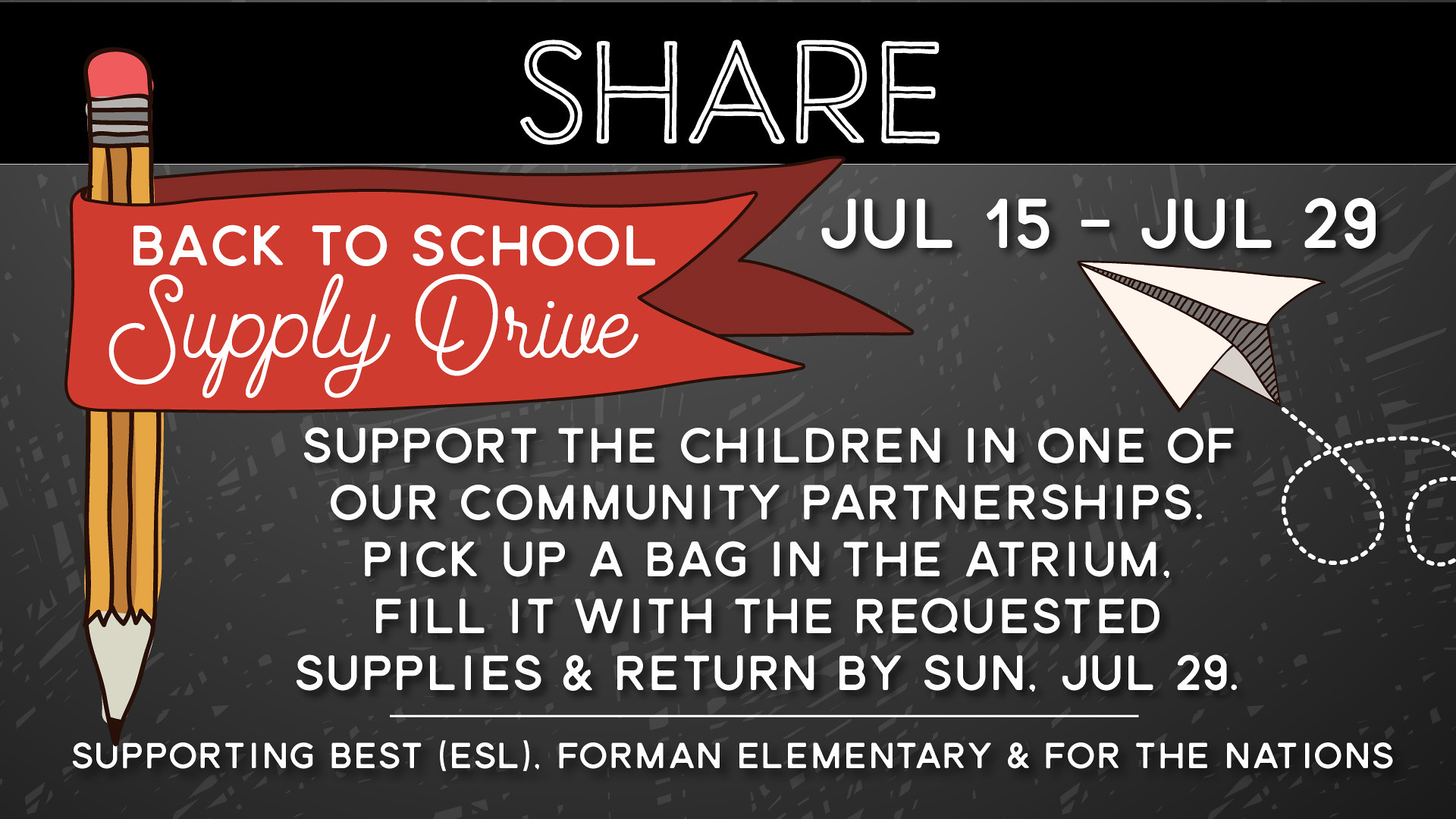The image is an advertisement for a back-to-school supply drive. At the top of the ad, set against a black background, the word "SHARE" is prominently displayed in white text. Below it, on the left side, there's a stylized sketch of a pencil pointing downwards, wrapped with a red ribbon that reads "Back-to-School Supply Drive." On the right side, there's an illustration of a paper airplane with a trail line. Above the airplane, the dates "July 15 - July 29" are clearly indicated. Additional white text on a gray background at the bottom of the ad instructs viewers to "SUPPORT THE CHILDREN IN ONE OF OUR COMMUNITY PARTNERSHIPS. Pick up a bag in the atrium, fill it with the requested supplies, and return by Sunday, July 29." The initiative aims to assist Best ESL, Foreman Elementary, and Fourth Nations. The design elements, including the text and illustrations, appear to be set against a chalkboard-like background.